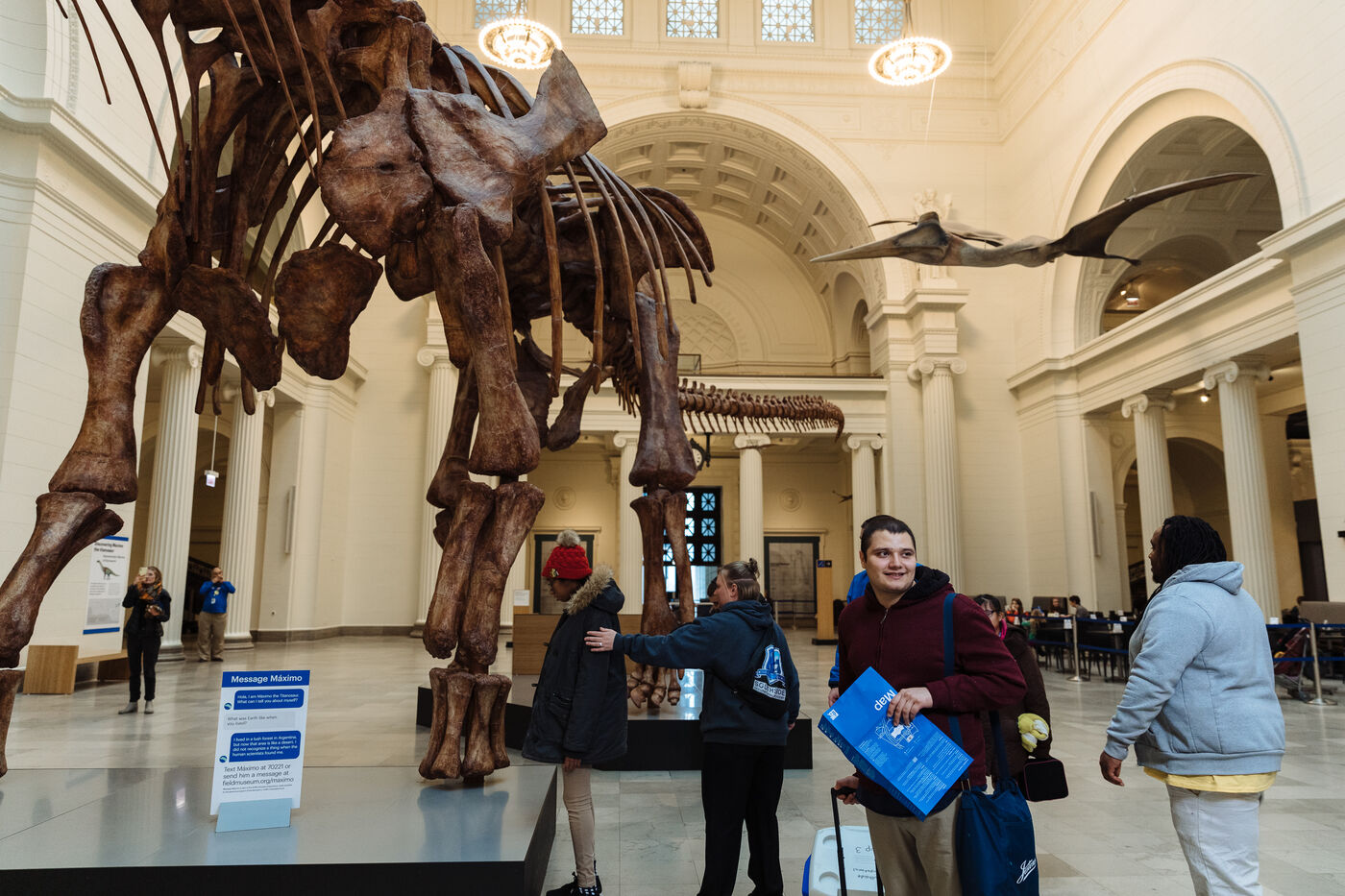The photograph captures an exhibit inside an ornate natural history museum, characterized by its very tall ceilings adorned with hanging chandeliers, high arched doorways, and columns on three sides of the room. The central focus of the image is a massive dinosaur skeleton, prominently displayed on a pedestal in the foreground. The dinosaur, dark brown in color, with only its large legs and a long tail visible, is elevated at least three or four times taller than the tallest person in the room. Suspended from the ceiling to the right side of the frame is a pterodactyl skeleton. 

Visitors are scattered throughout the spacious hall, including a young white man pulling a cooler and holding a dark blue map. Next to him stands a black man in a blue hoodie and white pants, looking up at the large dinosaur. Closely examining the dinosaur are two more visitors dressed in jackets; one of them wears a red hat. In the background, some benches and chairs occupy the space, with a few people seated. Near the pedestal supporting the dinosaur skeleton, a blue and white sign is present, though its text is not readable. The room’s vastness and architectural beauty provide a grand setting for this captivating fossil display.